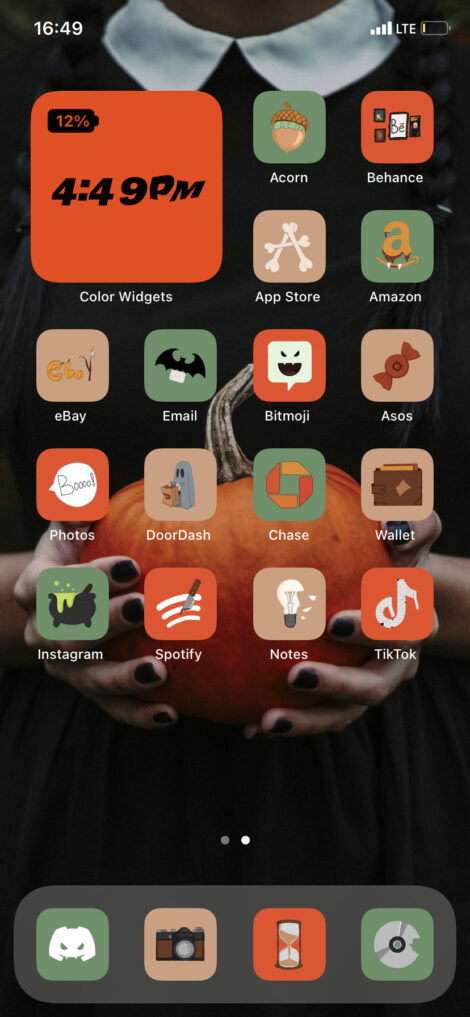Here is a cleaned-up and detailed caption for the image:

---

The screenshot from a cell phone displays the home screen background. At the top of the screen, the time reads 4:49 PM (1649). To the right, indicators show an LTE connection, a cell signal strength icon, and a battery icon with a small amount of yellow, indicating a 12% charge.

The background image features a muted green, "Peter Pan" colored sweater. The sweater-clad hands are holding an orange pumpkin with a prominently curved stem. Above the background image, there is a semi-transparent widget that displays the battery percentage (12%) and time (4:49 PM) in black text.

Below this widget are various application icons arranged in a grid. The apps visible include: 
- **Acorn**
- **Balance**
- **Behance**
- **App Store**
- **Amazon**
- **eBay**
- **Email**
- **Bitmoji**
- **Asus**
- **Photos**
- **DoorDash**
- **Chase**
- **Wallet**
- **Instagram**
- **Spotify**
- **Notes**
- **TikTok**

At the bottom of the screen, docked icons represent key features and tools: Phone, Messaging, Camera, and a Web Browser.

---